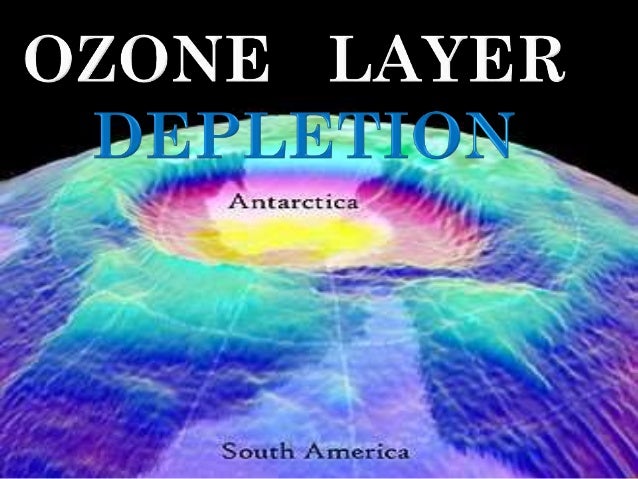The image is a detailed graphical representation of ozone layer depletion. It portrays a 3D rendering of the Earth, focusing on the Antarctic region. The Earth is colored thermally, with cooler areas in shades of blue and green, and hotter areas represented in yellow and red. At the center of the image, the continent of Antarctica is prominently displayed, appearing somewhat sunken to illustrate the extent of ozone depletion in that area. At the top of the image, bold white text reads "Ozone Layer," while directly below, "Depletion" is written in dark blue font. The middle section of the globe is labeled "Antarctica" in black text and at the very bottom, the label "South America" is visible, signifying the southern tip of the continent. The background of the image is solid black, which contrasts sharply with the colorful thermal map of the globe. This visual, reminiscent of a textbook illustration, occupies about two-thirds of the image from bottom to top, emphasizing the regions most affected by ozone layer depletion.